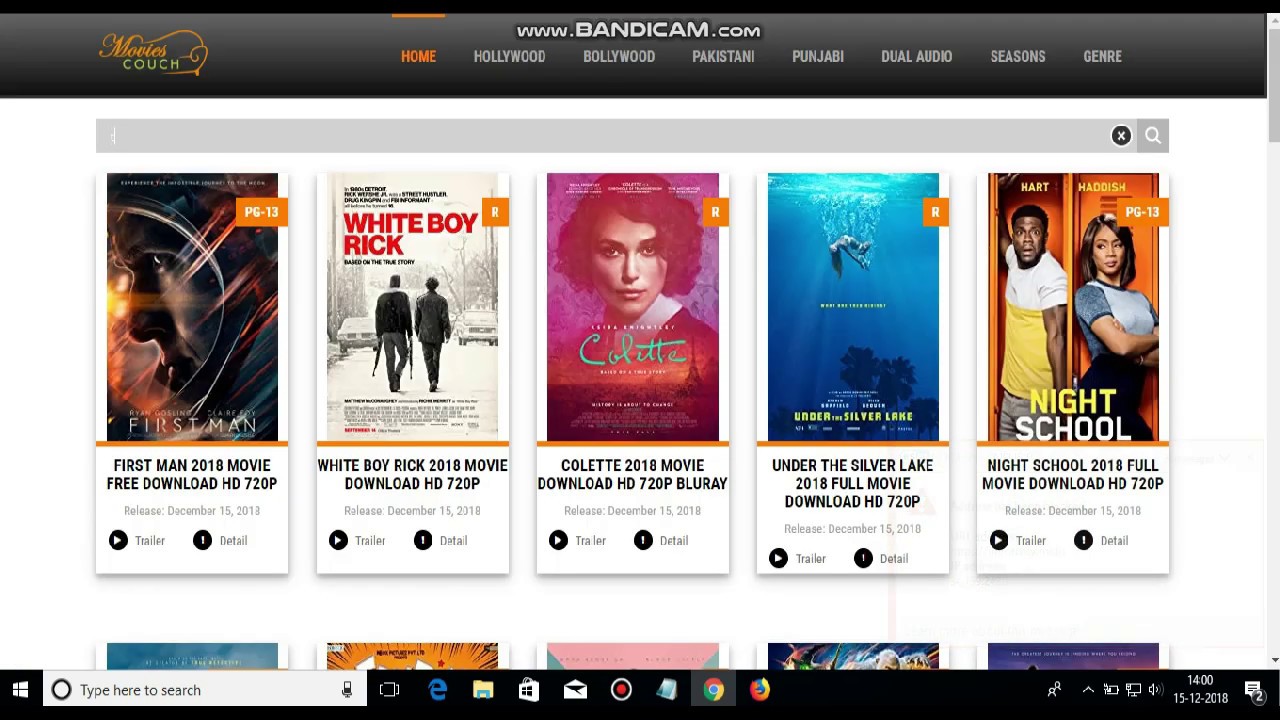The image displays a screenshot of the website Bandicam.com, which offers a variety of movies across different categories. The distinct sections available for browsing include Hollywood, Bollywood, Pakistani, Punjabi, Dual Audio, Seasons, and Genre, suggesting that it might cater to a diverse, possibly international audience rather than solely an American one.

Featured prominently on the website are several movie thumbnails. The first movie showcased is "First Man" (2018), depicting an astronaut against a striking backdrop. The next film is "White Boy Rick" (2018), shown in a black and white photograph that features a black man and a white man walking down the road together. Following this is "Colette" (2018), with an alluring image of a woman staring directly into the camera. Another featured film is "Under the Silver Lake" (2018), represented by an underwater scene. Lastly, "Night School" (2018) highlights Kevin Hart and Tiffany Haddish standing back-to-back.

Beneath these highlighted films, the website indicates there are more movie options available, although they are not visible in this specific image. The website offers further actions, such as watching trailers or obtaining more details about the movies.